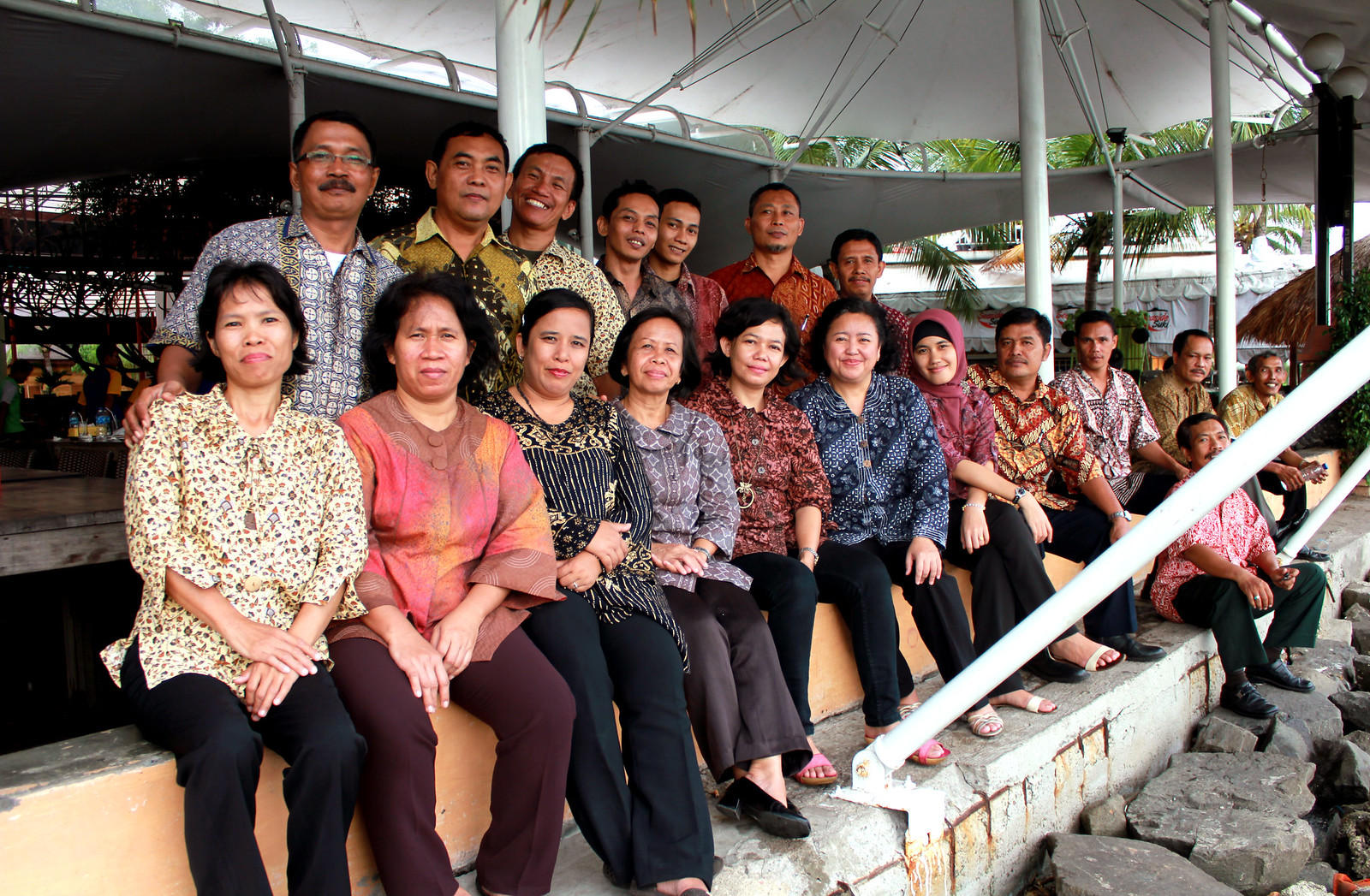This photograph captures a large group of approximately 19 people, likely an Asian family, sitting together under a spacious white tent canopy. The group, which includes both men and women across various age groups, appears to be outdoors in a tropical climate, possibly in the Philippines. They are seated on a low concrete wall, with some standing behind it. Notably, a man on the far left sports a mustache and glasses, while others in the group exhibit similar features, including dark black hair. The canopy they are under is supported by large cylindrical white poles, creating an open-air structure. In the background, there are signs of activity with other people walking around, potentially indicating a market or a resort-like setting, as additional tents and palm trees can be observed in the distance.